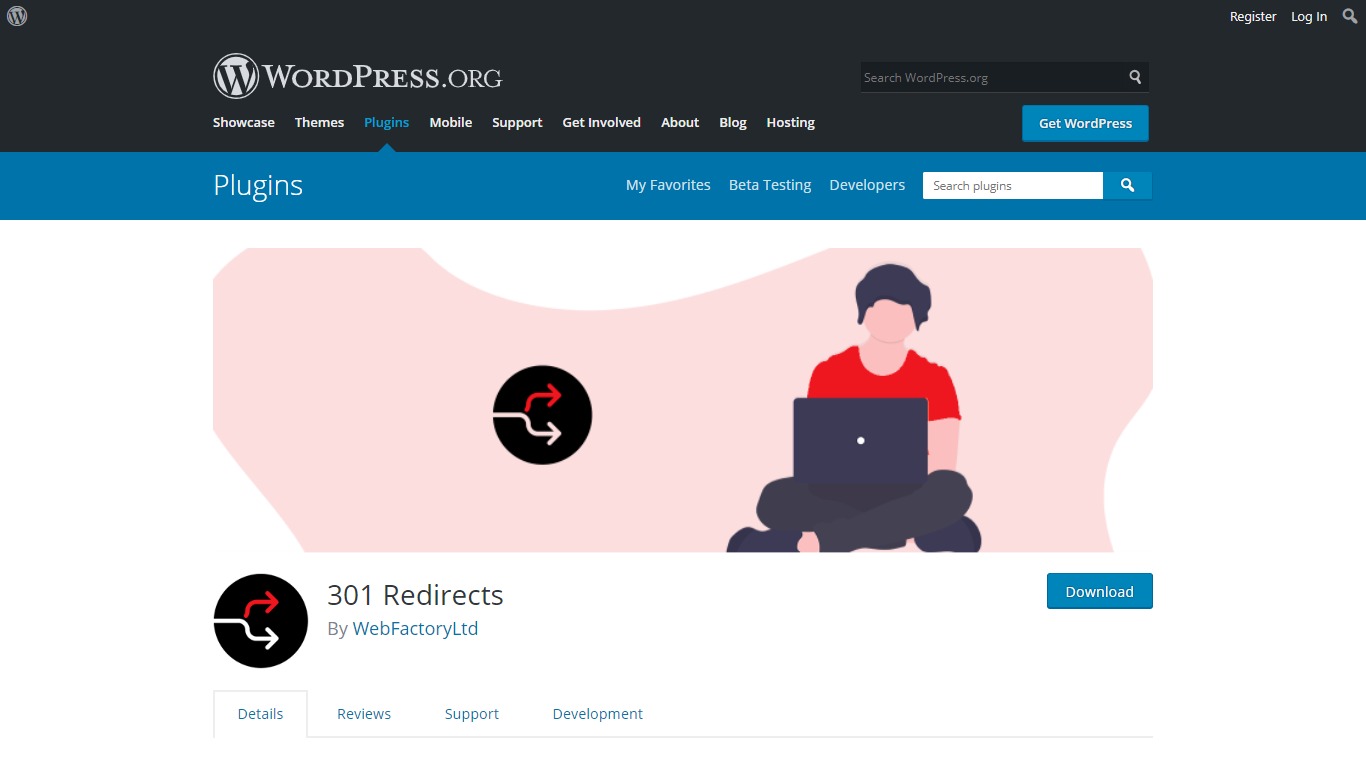The image displayed is of the WordPress.org website interface. The header section on the top right includes several navigation options such as "Register," "Login," and "Search" buttons. Adjacent to these buttons are additional menu categories including "Showcase," "Themes," "Plugins," "Mobile," "Support," "Get Involved," "About," "Blog," "Hosting," "WordPress," "Plugins," "My Favorites," "Beta Testing," and "Developers." Directly to the right of the navigation options is a search box, currently populated with the text "Search plugins."

As we move further down the page, there is an image of an individual using a laptop, situated comfortably on their lap. Below this image, the focus shifts to a plugin section featuring "301 Redirects" by WebFactory. Additional details provided include options such as "Details," "Reviews," "Support," and "Development," each presumably linking to further information regarding the plugin's specific aspects and user interactions.